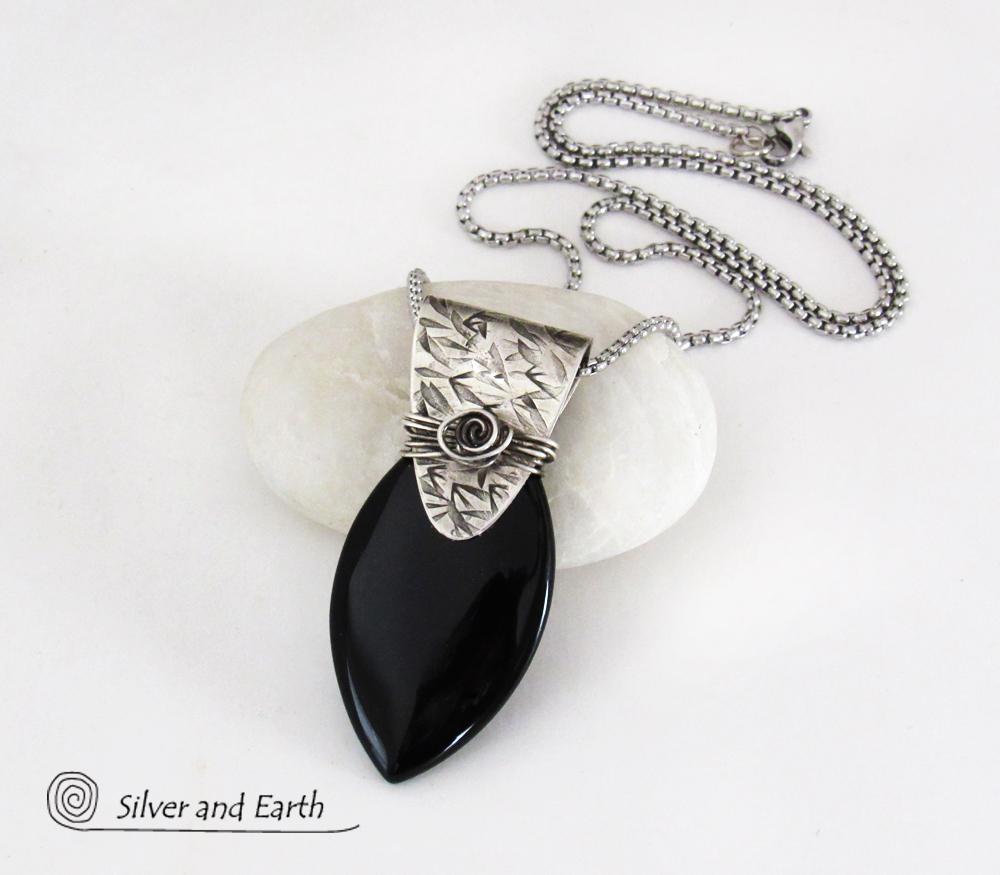The photo features an artistic advertisement for a necklace by "Silver and Earth." Set against a pearly gray background, the focal point is a striking silver chain with a thick, textured design. The centerpiece of the necklace is an elegant pendant: a teardrop-shaped, glossy black gem, possibly onyx, encased in a sleek silver setting. The pendant rests prominently atop a white stone surface, with its chain elegantly draped behind it. In the bottom left corner of the image, the brand name "Silver and Earth" is written in thin black letters, accompanied by a subtle, swirly logo. The overall composition and aesthetic suggest a high-quality, carefully crafted piece of jewelry designed to capture attention and exude sophistication.